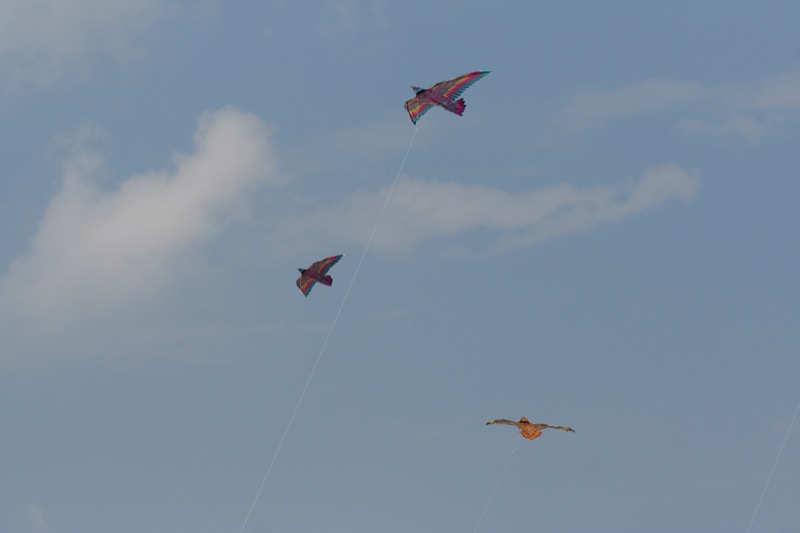Set against a medium light blue sky with puffy white clouds and some wispy clouds concentrated in the center and right, three vividly colorful kites shaped like birds are soaring high above. Two of these kites, nearly identical, showcase bodies of purplish blue with black stripes, their wings adorned with rainbow patterns that transition from bright blue to hot pink and yellow. These birds also sport tail feathers of hot pink and small colorful plumes on their heads. The third kite, differing slightly, features an orange body with similarly striking rainbow wings. Their delicate strings descend from the kites, swaying gently as the wind guides these dazzlingly vibrant bird-shaped kites across the sky. In the bottom right corner, an additional string can be seen, hinting at another bird just out of the frame. The overall scene captures a delightful and lively display of airborne colors and whimsical design, reminiscent of nature’s birds but amplified in a spectrum of hues.